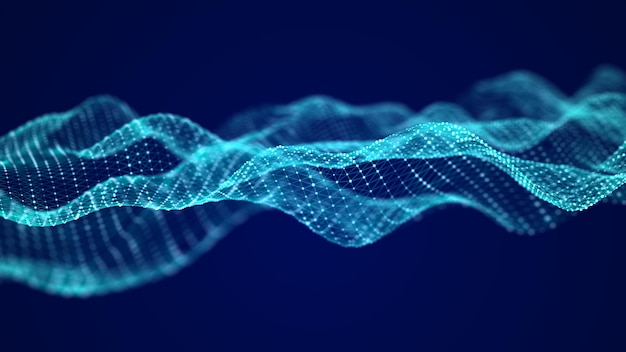The image is a detailed representation of a neon blue, zig-zag patterned mesh on a dark blue background. The fluorescent blue grid has a wavy texture and appears to twist into a shape reminiscent of DNA sequencing. The grid pattern overlaying the dark blue backdrop creates an illusion of mountains and valleys, akin to a radar map or a layered, three-dimensional mesh. The fabric-like structure, resembling plastic cloth with clear fluorescent light blue dots, flows side to side, giving it a dynamic, wave-like quality. It blends the aesthetics of DNA helixes, radar maps, and a textured grid to form a complex and mesmerizing visual.